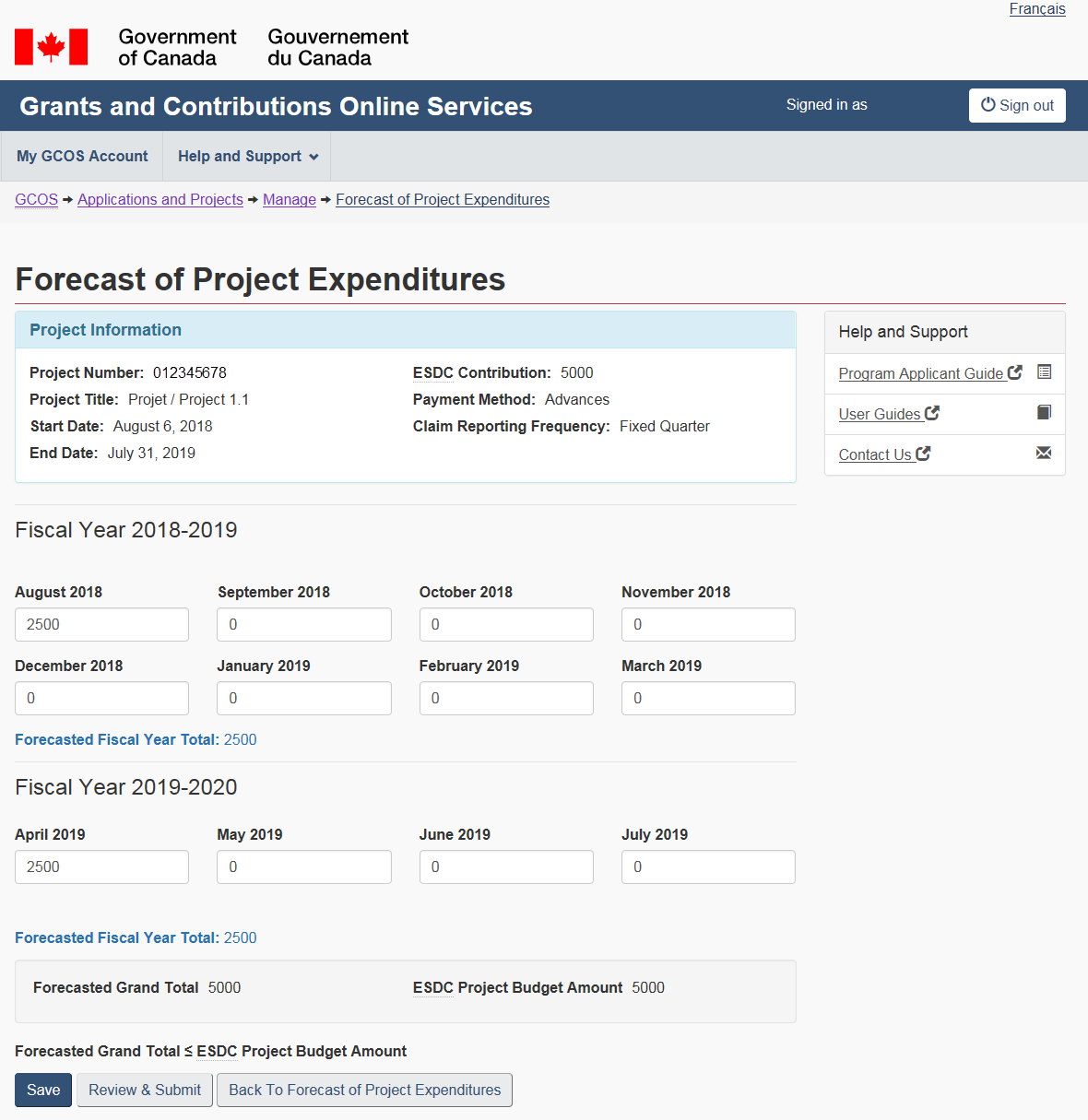This is a detailed screenshot of a Canadian government website. At the top left corner, there is a Canadian flag, identifiable by its red stripes on the sides and a white center featuring a red maple leaf. Next to it, the text "Government of Canada" is displayed, followed by the French equivalent, "Gouvernement du Canada." At the top right, the word "Française" indicates a language option for French.

Beneath the Canadian flag, a blue bar contains white text stating "Grants and Contributions Online Services." To the right, it shows the phrase "Signed in as," though the specific user's name is obscured. There is also a white "Sign out" button on the top right of this bar.

Directly below the blue bar, the interface provides navigation links labeled "myGCO's account" and "Help and support." The main content area of the page features a title that reads "Forecast of Project Expenditures," under which a section titled "Project Information" is displayed.

The "Project Information" section details the following:
- Project Number: 012345678
- Project Title: Project 1.1 in Project
- Start Date: August 6, 2018
- End Date: July 31, 2019